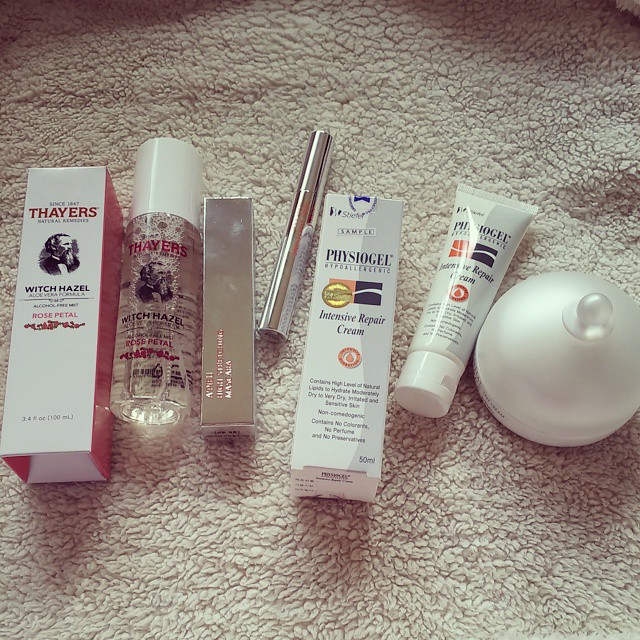A detailed and descriptive caption for the image could be:

On a well-worn, white sherpa blanket, softened by numerous washes, several beauty products are meticulously arranged. Dominating the scene is a red and white box adorned with elegant black writing that reads, "Since 1847, Thayer's Natural Remedies." The box prominently advertises their Rose Petal Witch Hazel product, complete with decorative banners at the bottom. Beside the box lies the extracted product: a clear bottle with a pump and mist dispenser. Next to this, a silver box with red writing catches the light, making it difficult to decipher, but its contents—a sleek, silver tube resembling a mascara—are placed nearby. Completing the assortment is a box labeled "Physiogel Intensive Repair Cream." The predominantly white and gray packaging is accented with blue and red, and just beside it rests the extracted product. Adding a touch of elegance to the arrangement is a circular object with a handle, which appears to be glass, subtly reflecting the soft ambiance of the worn sherpa fabric.